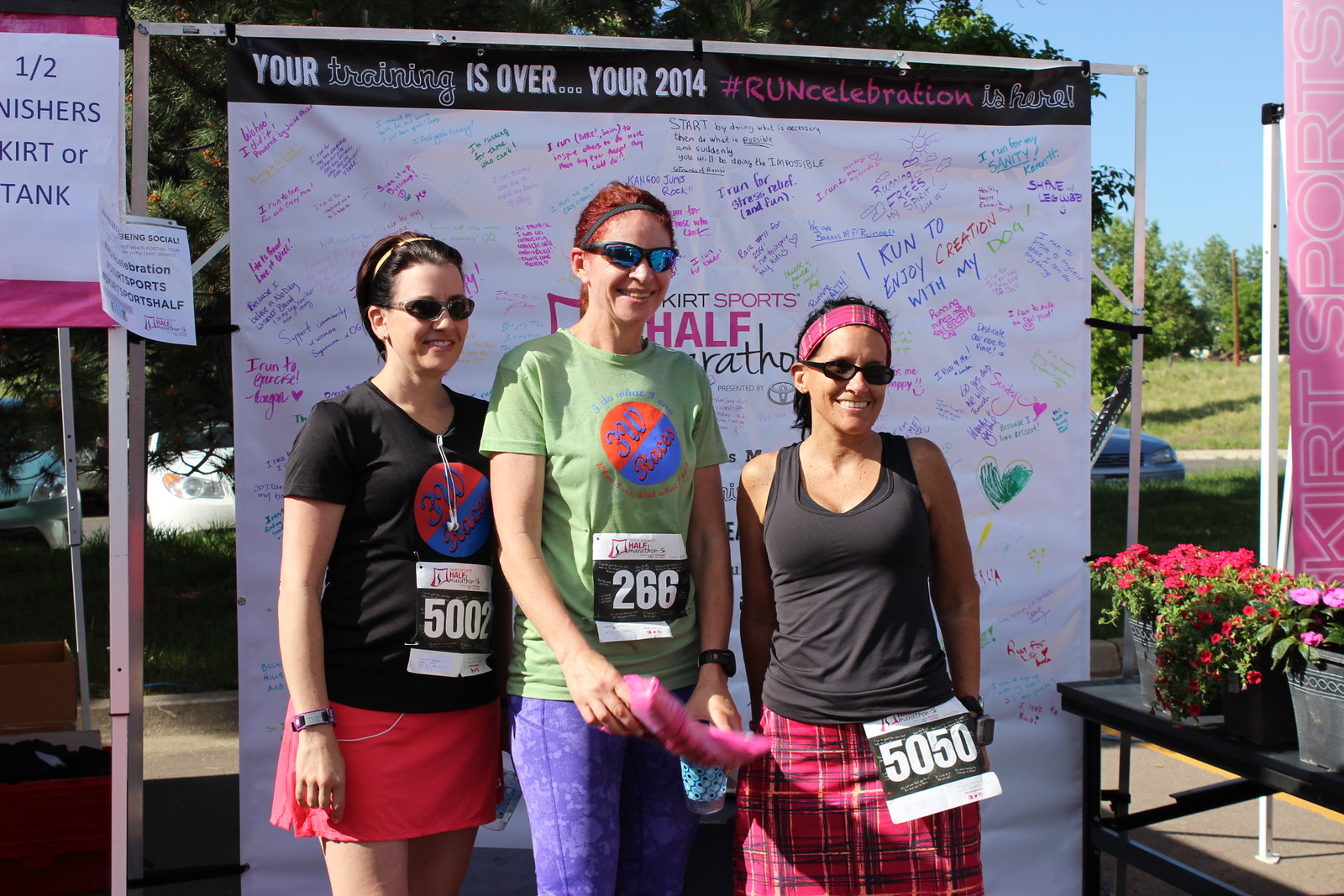This color photograph captures three women who appear to have just completed a marathon, standing together in front of a celebratory banner that reads, "Your training is over, your 2014 #Run Celebration is here." The banner, adorned with various signatures and messages in multiple ink colors, emphasizes their accomplishment. From left to right, the first woman has dark hair and is wearing a black t-shirt with the bib number 5002 and a short red running skirt. The tall red-haired woman in the middle is dressed in a light green t-shirt and purple exercise pants, with the bib number 266. The last woman, who is short with long dark hair, sports a pink bandana, a black athletic tank top, and a pink plaid athletic skirt; her bib number, 5050, is pinned to her skirt. The photograph, taken outdoors, also features a small black table with potted pink and purple flowers blooming on the right-hand side, adding a vibrant touch to the scene. Behind the women, trees are visible, completing the lively and triumphant atmosphere of this marathon finishers' photo.